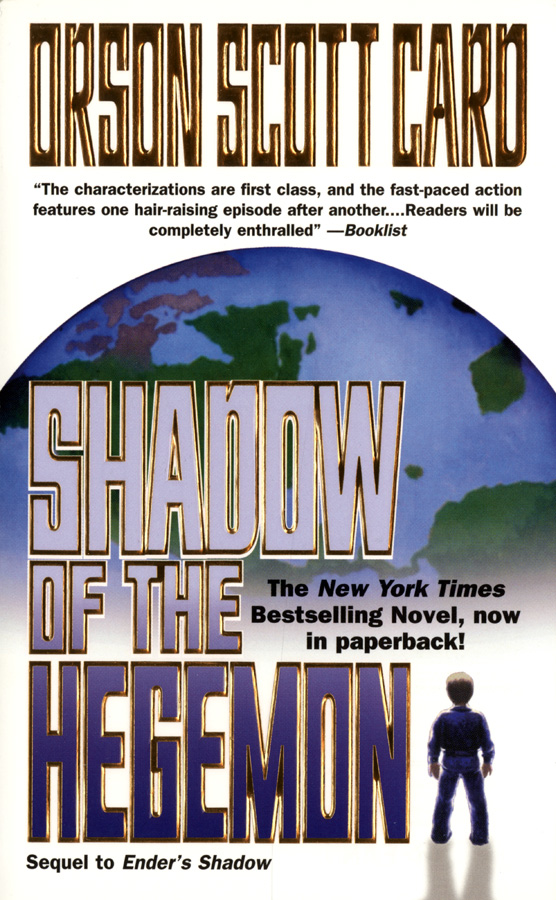This image is a promotional poster for the book "Shadow of the Hegemon" by Orson Scott Card. At the top, the author's name is displayed in highly stylized black text on a white background, making it slightly difficult to read. Below, in clean sans-serif print, is a quote in black text: "The characterizations are first-class and the fast-paced action features one hair-raising episode after another... Readers will be completely enthralled." This quote is attributed to Booklist. 

The white background continues down the image but is interrupted by an arched graphic. At the top of this arch is a gradiented depiction of a globe, which melds into the white background at the lower third of the image. Overlaying this globe is the title of the book in light blue text outlined in black and then in white: "Shadow of the Hegemon," with "Shadow" at the top, "of the" in the middle, and "Hegemon" in tall letters at the bottom. To the right of "Hegemon" is a stylized, clay-model-like figure of a male character casting a long shadow.

Beneath "Hegemon," in black italic sans-serif text, it reads: "Sequel to Ender's Shadow." To the right of "of the," over the gradiented globe, there is more black italic sans-serif text that states: "The New York Times bestselling novel, now in paperback!"